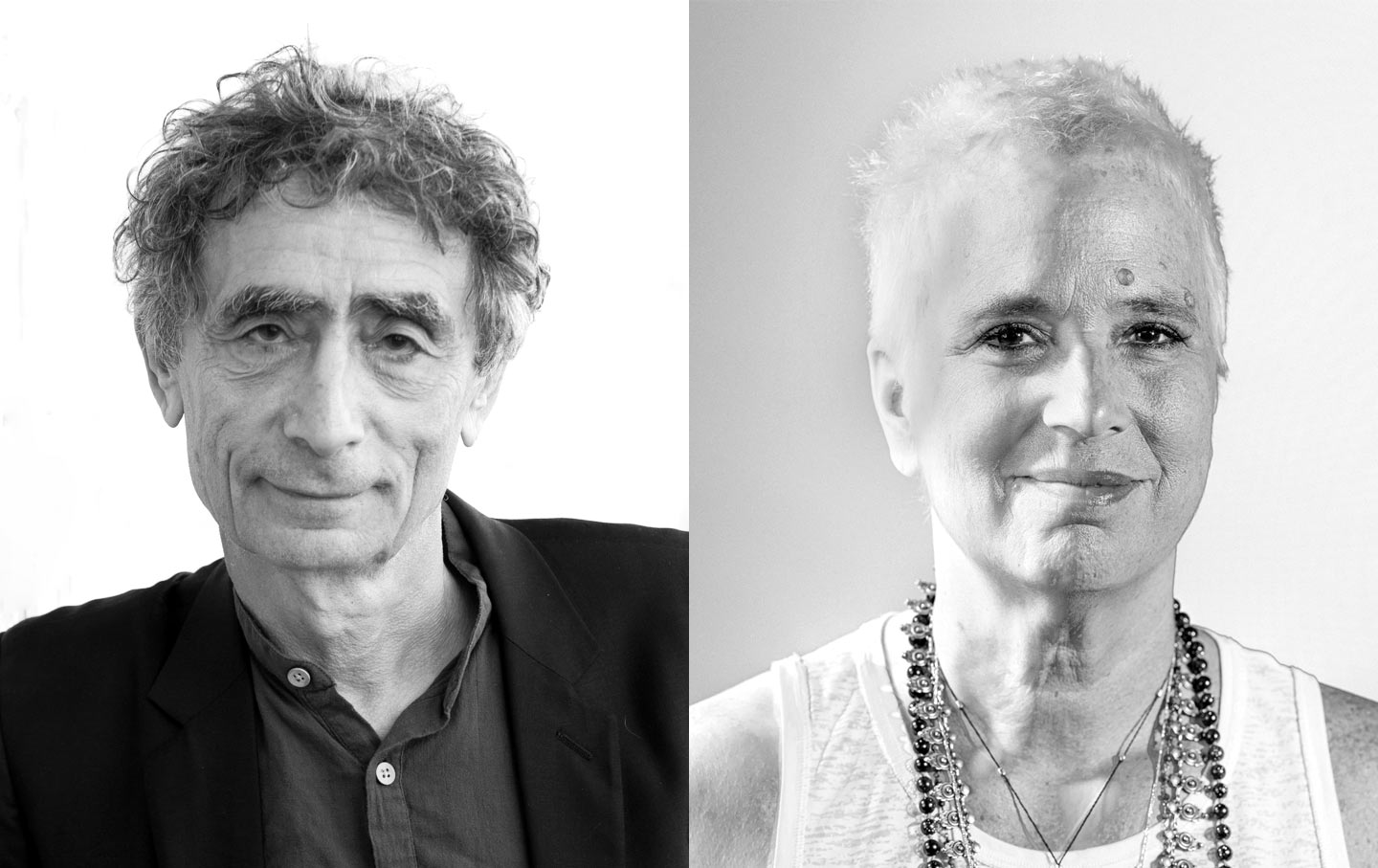The image features two black-and-white photographs placed side by side. The photograph on the left portrays an elderly Caucasian man with short, wavy, salt-and-pepper hair. He has very bushy eyebrows and prominent eye bags, suggesting a tired appearance. His eyes appear droopy and thick-lidded, and though he has slight smile lines, his expression is more neutral with a closed mouth. He is dressed in a dark suit jacket over a dark button-up shirt, against a solid white background.

The photograph on the right depicts a middle-aged Caucasian woman with extremely short, almost shaved, platinum blonde or gray hair. She is smiling with a closed mouth, revealing dark eyes and a friendly demeanor. Above her left eyebrow, she has two noticeable moles. She is adorned with multiple necklaces, including beaded and metallic ones, and she wears a sleeveless white tank top. Her image has a light gray background, complementing her bright, cheerful appearance.